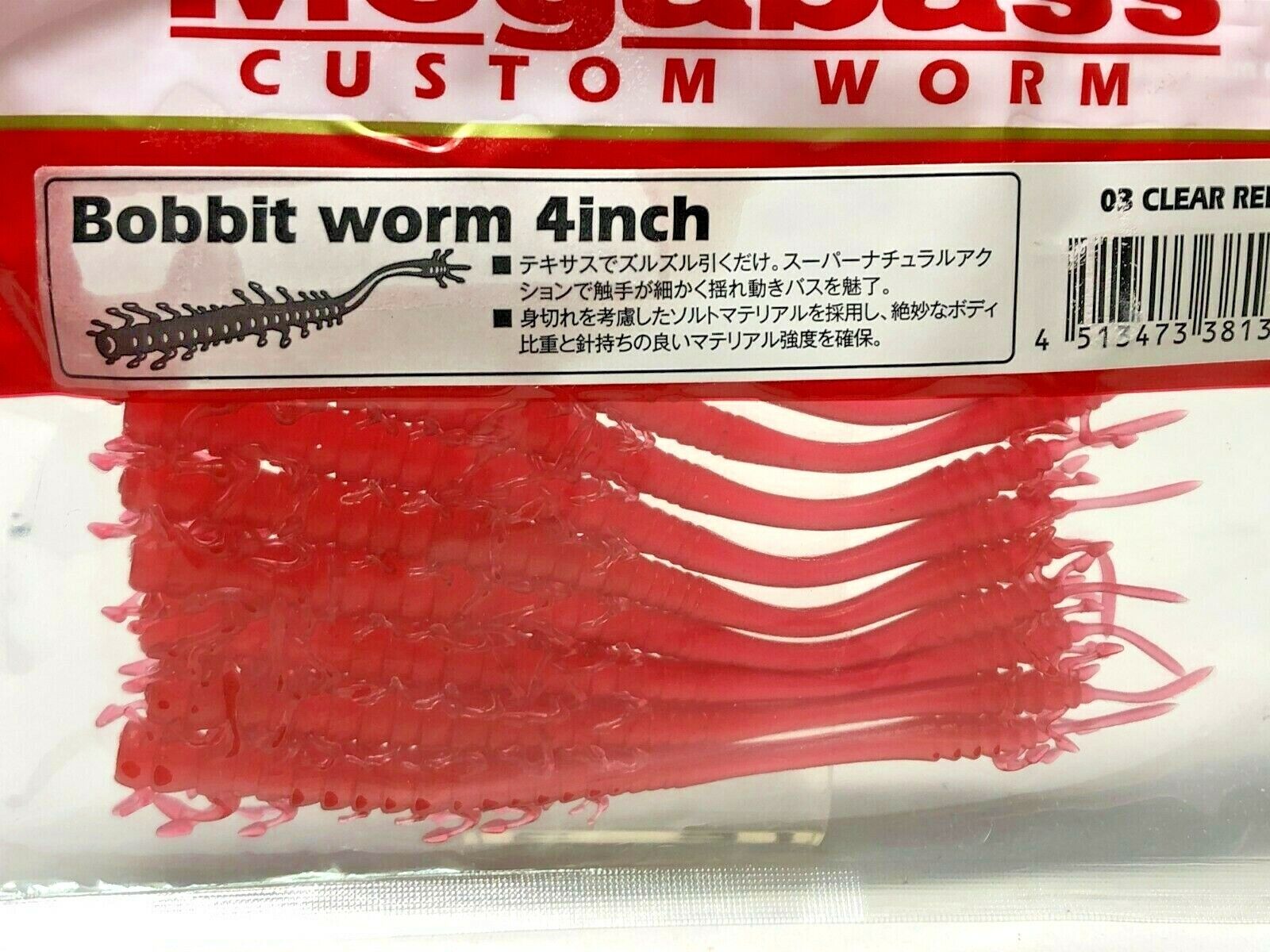This photograph captures the detailed packaging of a fishing bait product prominently featuring both Japanese and English text. At the top, partially cut-off red text reads "Custom Worm," followed by black text that clearly states "Bobbitt's Worm 4 inches." The package includes a visual example of the bait in black and white. To the right, the text "03 Clear" is visible, though the following characters are cut off. Additionally, there are two square bullet points with Japanese text. Below this section, there's a barcode with the number 45134733813, though the rest is partially obscured. Attached to the bottom of the packaging is a clear plastic bag containing at least nine red Bobbitt worms, making the overall package both informative and visually representative of the product.